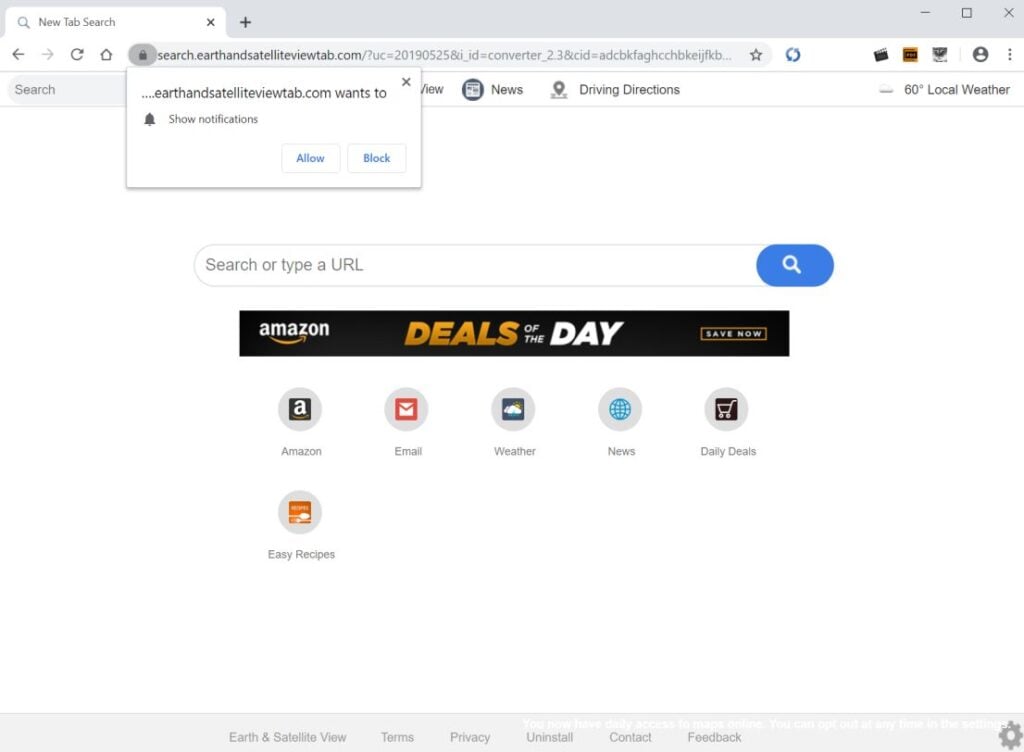This screenshot captures a detailed view of a website interface, showcasing various features and elements. At the top, a light gray background sets a neutral tone. Immediately below, a search bar is prominently displayed. This search bar, with a blue background and a magnifying glass icon, includes the placeholder text "Search or type a URL," signaling its function as a search engine tool.

In the top left corner of the image is a notification prompt from "earthandsatelliteview.com," offering the options to "Allow" or "Block" notifications, each option highlighted in blue text.

Beneath the search bar is a black advertisement banner promoting "Amazon Deals of the Day," where "Deals" is highlighted in yellow, "of the day" in white, and the call-to-action "Save Now" is prominently featured.

Following this, there are six application icons arranged in a grid against a white background, each encapsulated in a light gray circle. From left to right, the icons represent:
1. Amazon
2. Email
3. Weather
4. News
5. Daily Deals
6. Easy Recipes

Finally, at the bottom of the screenshot, the interface provides six navigational categories listed in a plain text format: Earth and Satellite View, Terms, Privacy, Uninstall, Contact, and Feedback. The bottom right corner features a settings icon symbolized by a gray gear, providing access to additional configuration options.